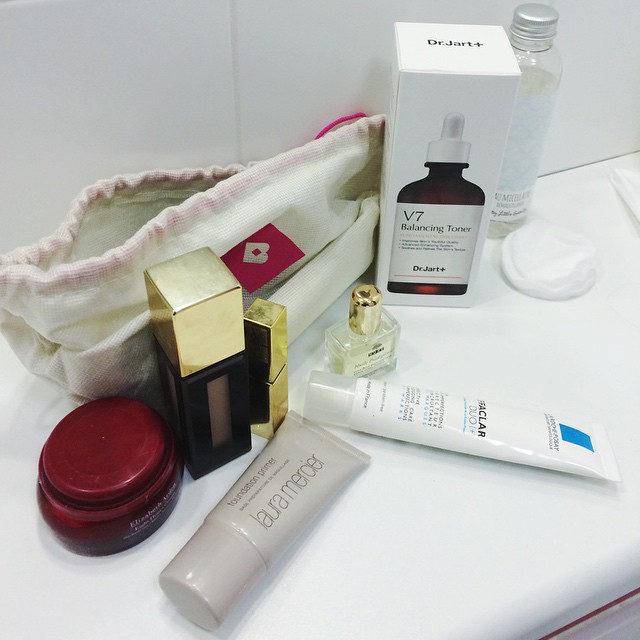On a pristine white countertop, a curated collection of beauty products is meticulously arranged. Prominent among them is Laura Mercier's gray tube of primer, exuding an air of sophistication. Next to it, Roche's nourishing face lotion stands ready for application, its sleek packaging promising hydrated skin. An unopened box of V7 Balancing Toner adds an element of anticipation, suggesting the promise of perfectly balanced skin with its first use.

Alongside these, evidence of a recent skincare routine is found in a used cotton pad. Two lipsticks, one with a striking red casing identifying it as Elizabeth Arden, hint at possibilities for glamorous looks. Completing the ensemble is a clear perfume bottle adorned with a gold cap, ready to leave a lingering scent.

Amid these beauty essentials lies a distinctive white case made from waffle-textured material. It features a pink string closure and a pink square with a 'B' monogram, embellished with a tiny diamond at its center. This charming case seems to be a protective home for the beauty tools when not in use, adding both function and style to the countertop's display.